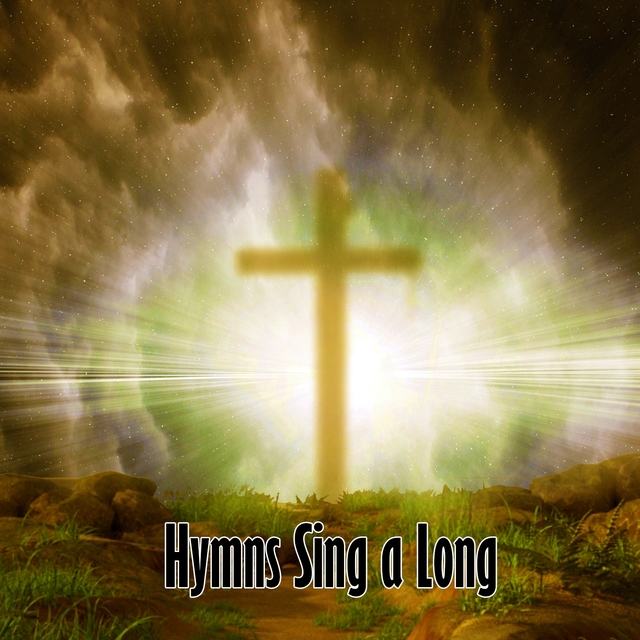The digitally created image, likely intended for an advertisement, church bulletin, calendar event, or album cover, features a vivid and detailed outer space scene. The background showcases an off-black, starry night sky with scattered stars, overlaid by a nebulous cloud that transitions from a greenish-yellow center to white and pinkish hues outward. Dominating the center of the image is a luminous cross, colored mustard yellow, with radiant beams of light emanating in all directions, symbolizing a divine presence. Below this celestial display, the foreground depicts an earthy ground with sparse grass and rocks. Across the lower portion of the image, the black text "hymns sing along," highlighted by a yellow or white border, indicates the image's purpose, summarizing its religious orientation while remaining generically spiritual enough for varied denominations.